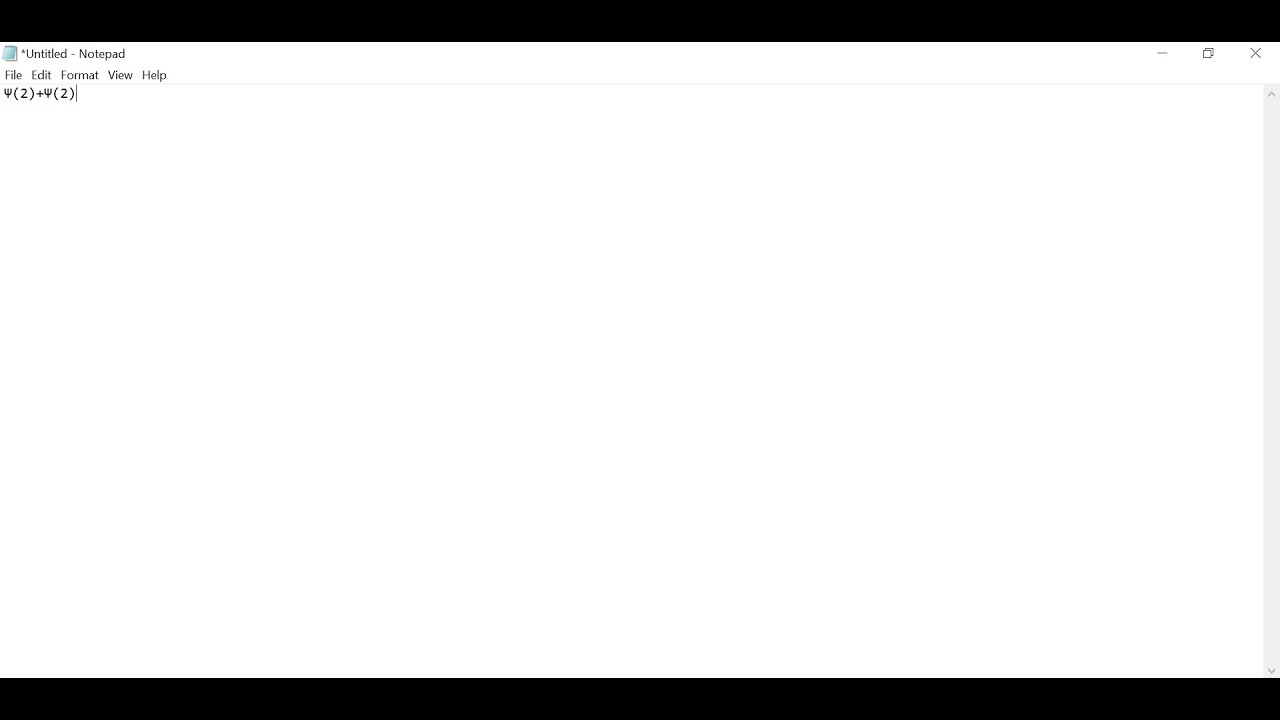The image depicts a screenshot of a Notepad window open on a computer screen. At the very top, a black title bar displays the text "Untitled - Notepad" alongside the minimize, maximize, and close buttons. Below the title bar, there is a menu bar with the options: File, Edit, Format, View, and Help. In the main body of the Notepad window, the text "epsilon (2 + 2)" is typed out. The Notepad interface is distinctly simple with a white background and plain black text, characteristic of the default Windows application.